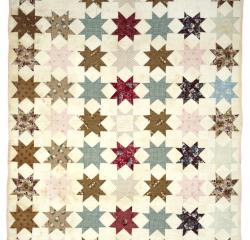This detailed illustration depicts a section of quilt-like cloth characterized by a geometrically patterned grid of eight-pointed stars against a cream background. Arranged in a meticulous, repeating pattern, the stars line up in seven vertical rows and eight horizontal rows. The star shapes exhibit a muted color palette that includes shades of black, olive green, light green, dark red, light gray, dark gold, blue, and light pink. Each color alternates as you move across the rows, creating a rhythmically subdued visual effect. The overall appearance is soft and nothing particularly stands out, making the design look balanced and consistent. Despite its intricate design, the object maintains a two-dimensional, flat look—evoking imagery of a tablecloth, quilt square, or some similar cloth-like material. The stars, whether gold, copper, red, blue, or gray, all share the same shape and size, reinforcing the symmetrical grid structure of the entire piece.